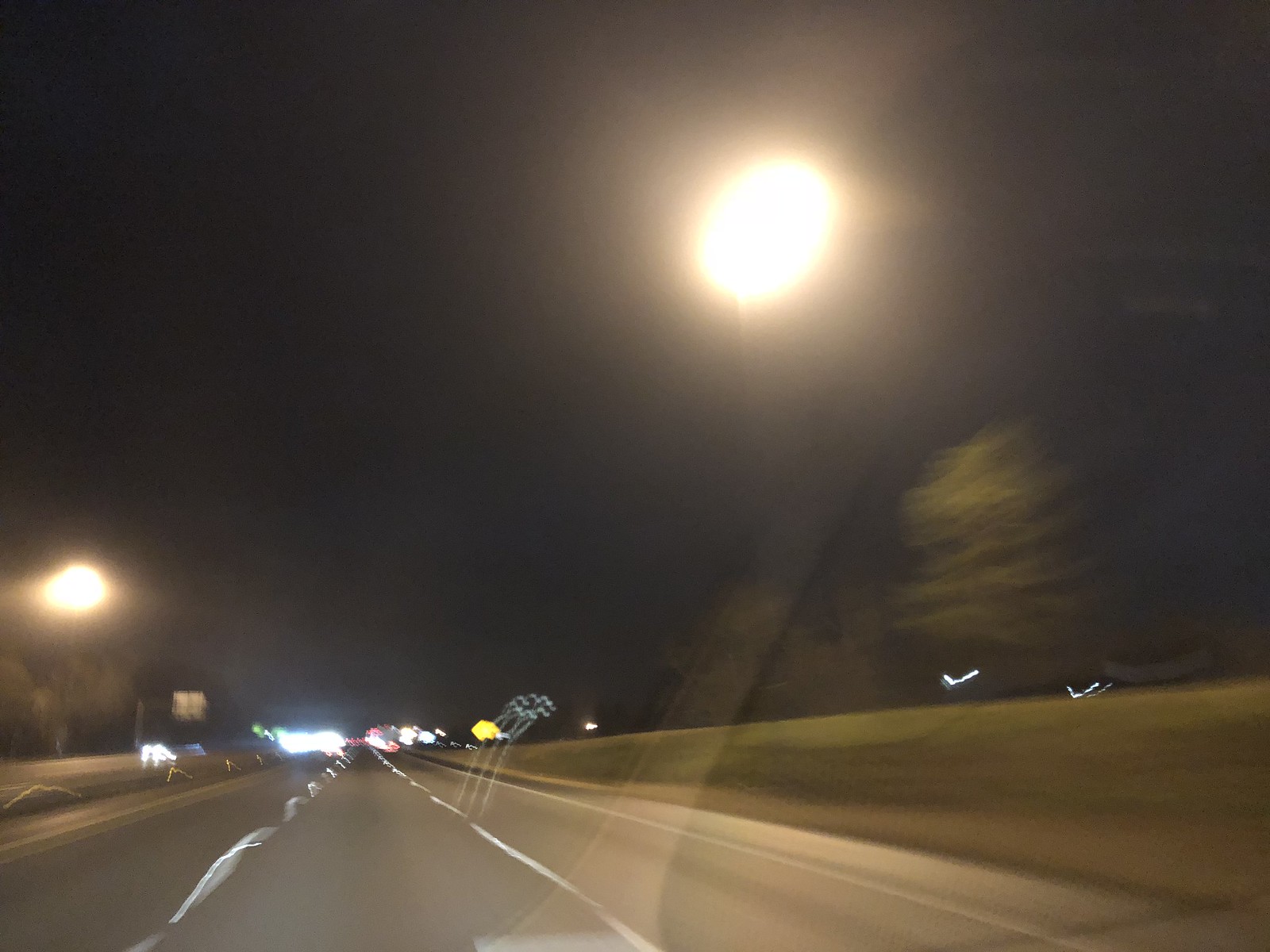This is a very blurry photo taken at night on a highway, likely from a moving car. The image is out of focus, capturing the streaky motion of the vehicle and surroundings. The sky is pitch black, devoid of stars or clouds, dominated by two bright orbs that appear to be glares from the streetlights. The highway is a multi-lane road, with the bottom left of the image showing streaks of headlights and taillights indicating traffic in both directions. The road is bordered by grass and trees, particularly on the left, where there are also streetlights. A reflective hint of the car's window can be seen, alongside a yellow street sign towards the top left of the photo. The overall scene appears wavy and blurred due to the motion, contributing to the abstract quality of the nighttime highway image.